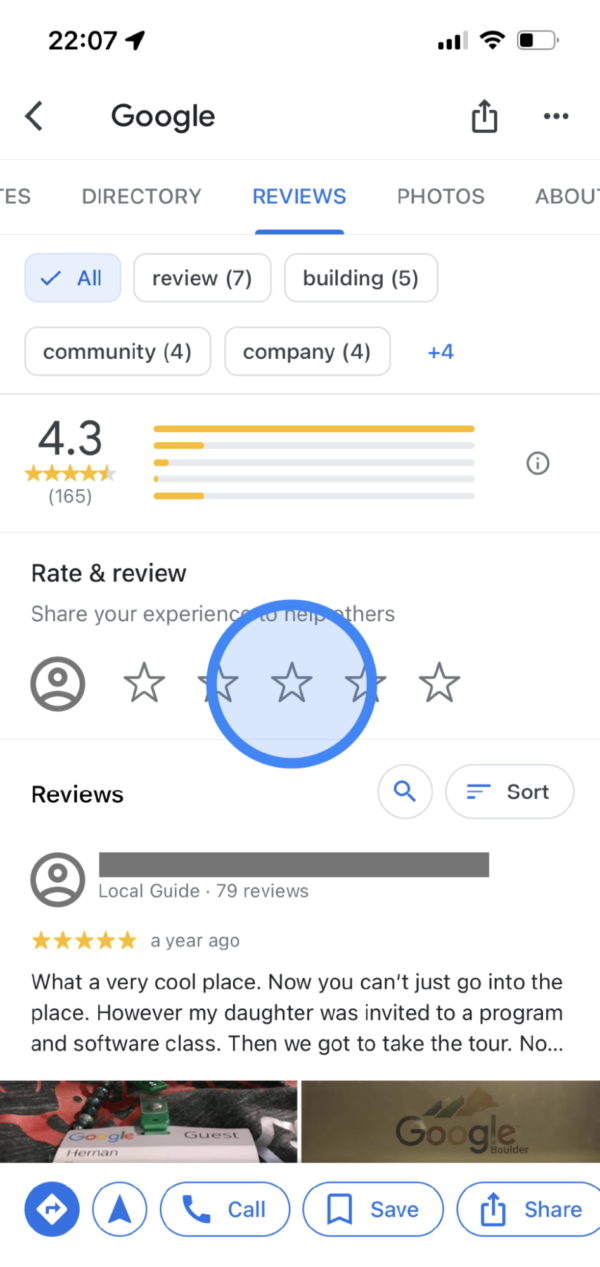The image depicts a smartphone screen displaying a Google search results page. The time indicated at the top of the phone is 22:07, and the battery icon shows less than half charge, while the Wi-Fi connection is strong. At the very top, the Google logo is visible alongside a download icon and a three-dot menu indicating additional options. 

The website displayed partially shows the word starting with "ES," which seems to be truncated. Below that, navigation tabs labeled 'Directory,' 'Reviews,' 'Photos,' and 'About' are visible, with the 'Reviews' tab currently active and underlined in blue. The filter box labeled 'All' is highlighted in light blue and marked with a check.

The page features a summary section indicating the site has a 4.3-star rating out of 165 reviews, with categorized reviews displaying 7 for 'Building,' 5 for 'Community,' and 4 for 'Company.' An invitation to rate and review is extended to users, with the text encouraging them to share their experiences to assist others. There's an emphasized, blue-rimmed circle around the third star, perhaps suggesting an interactive element for rating.

Beneath this summary, a review from a 'Local Guide' with 79 reviews is highlighted. Posted a year ago and rated five stars, the review reads: "What a very cool place. Now, you can't just go into the place. However, my daughter was invited to a program, a software class, then we got to take the tour..." The review abruptly ends there.

To the right of the review text is a faintly shaded "Google" image, while to the left, a partially visible image of a book is shown.